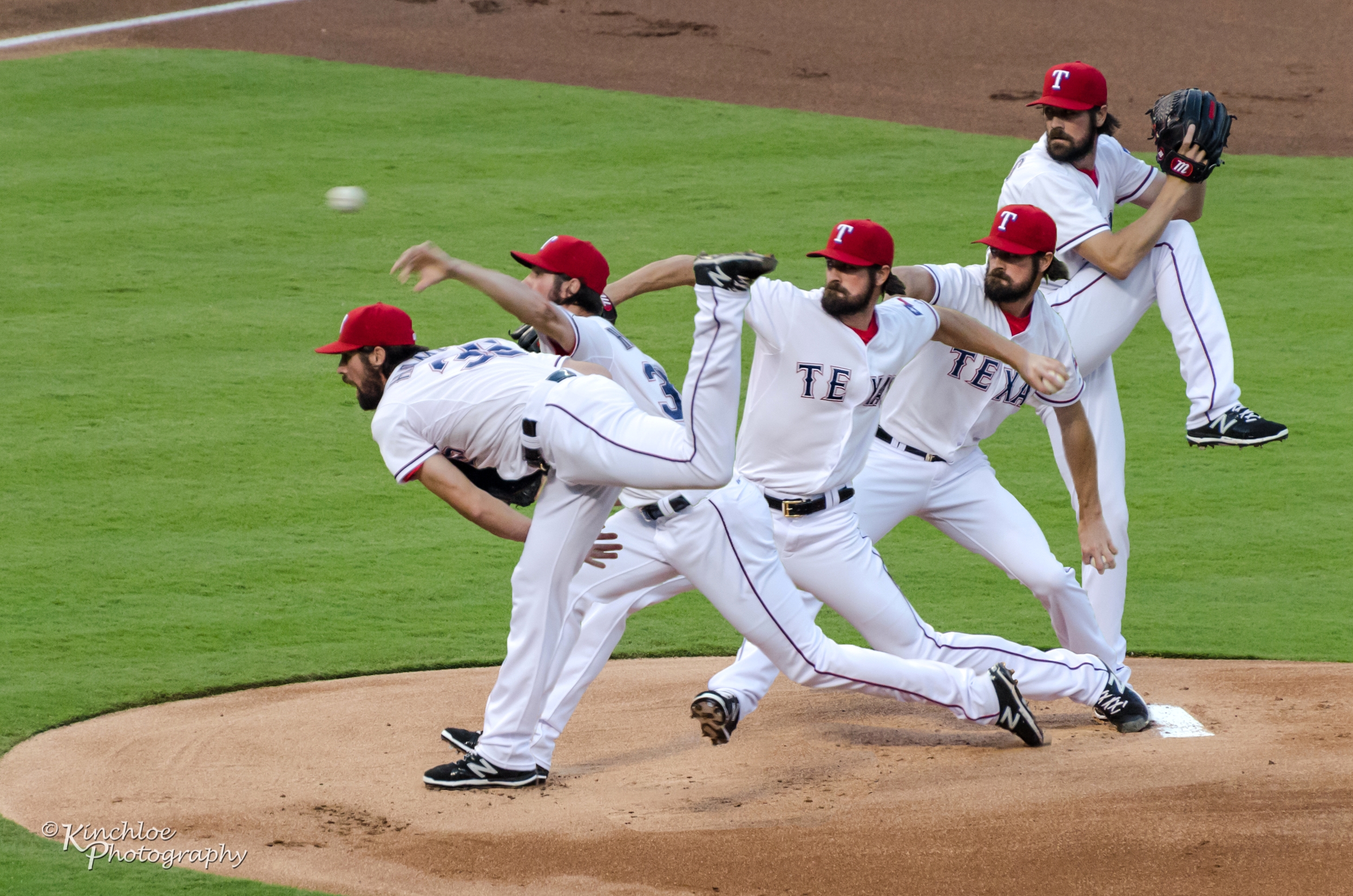The image is a professionally captured, composite photograph of a single baseball player, a white male with long dark hair tied in a ponytail and a thick beard, showcasing five sequential stages of him pitching a baseball. The player is dressed in a pristine white uniform with "Texas" emblazoned on the front, a red undershirt visible beneath. He dons a red and white baseball cap with a prominent white "T" on the front, black sneakers marked with a white "Z" or "N," and a black belt. The setting is an outdoor baseball field, clearly depicted with green grass and brown dirt. The sequence starts from the left, showing him poised with his leg lifted and ball in his mitt, progressing through to the final action of throwing the ball, now visible out of focus in mid-air. This image effectively captures the dynamic motion of the pitch, emphasizing the player's focus and athletic form.